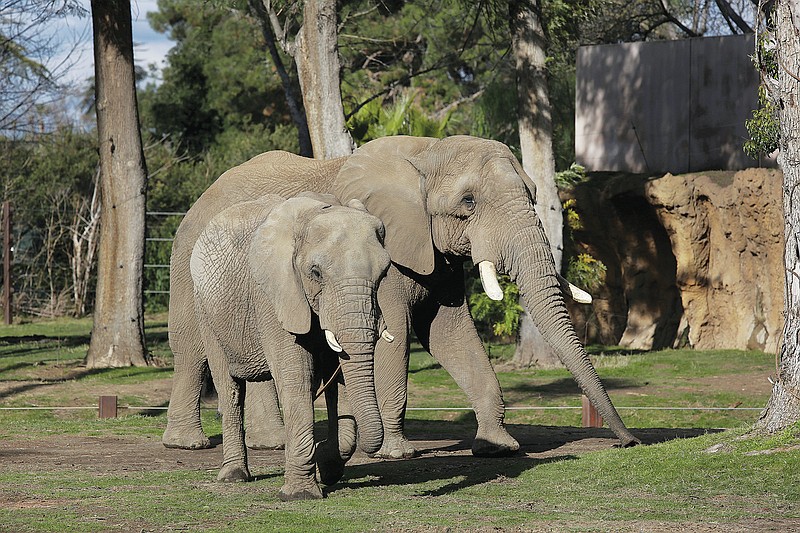The image captures a close-up view of two sandy brown elephants walking side-by-side. The larger elephant, likely the mother, has prominent tusks and is accompanied by a smaller, younger elephant. Both elephants have their trunks extended in front of them. They are moving across a flat, matted-down surface with very short grass. Surrounding them are large, green trees, hinting at a natural setting, but visible signs such as square wooden pegs with white string and a fence between the trees suggest they are in a nature preserve rather than the wild. The clear blue sky with scattered clouds completes the scenery in the background.